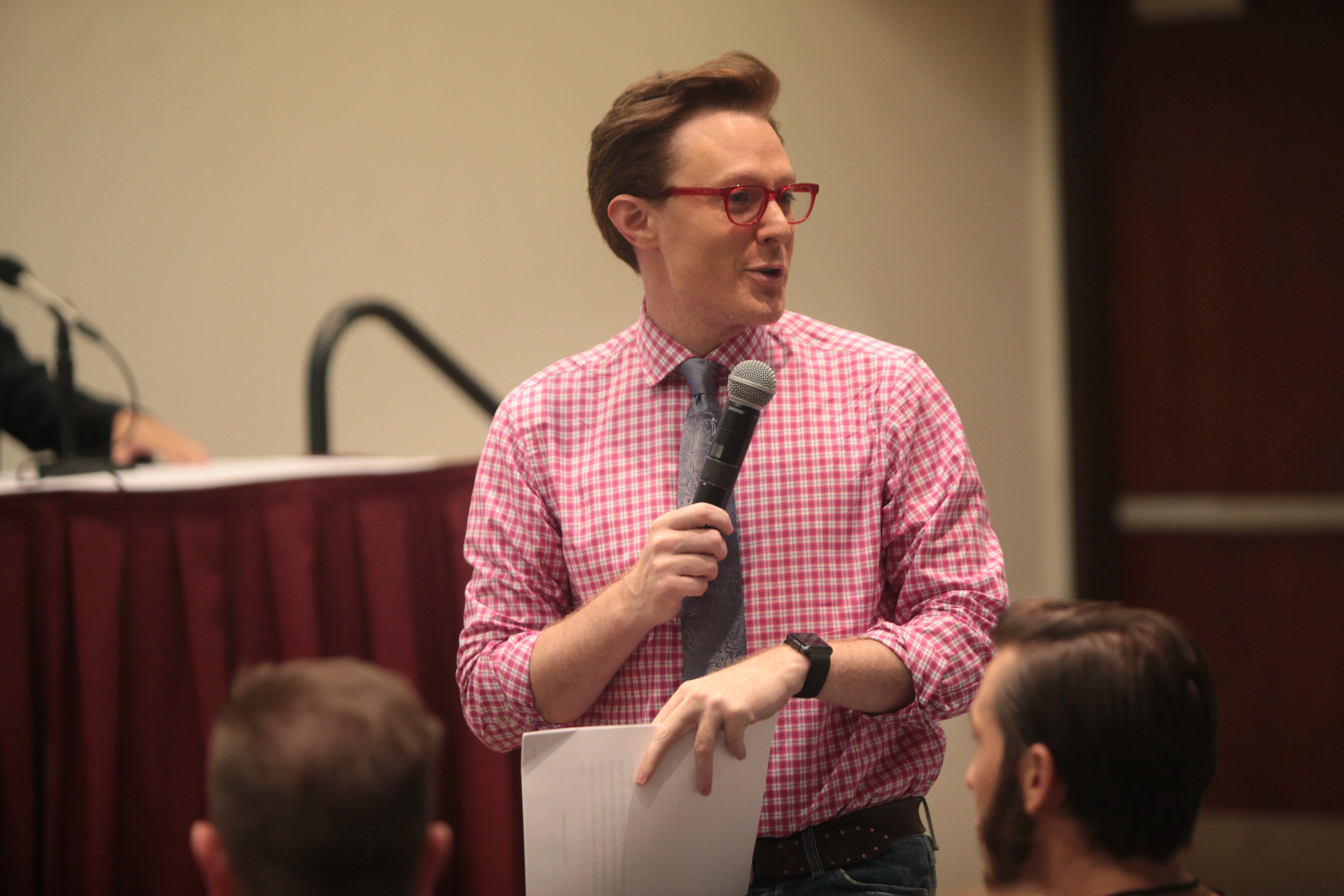The photograph showcases a man, centrally positioned, speaking into a microphone while holding a stapled stack of papers in his other hand. He is wearing a distinctive red and white checkered dress shirt, which evokes a picnic tablecloth pattern, tucked into blue jeans secured with a belt. His ensemble is complemented by a black watch on his wrist, a gray tie around his shirt, and red translucent glasses that give off a slightly nerdy, retro vibe. His medium-length, orangish-brown hair is neatly swept back. Surrounding him, there are a few audience members visible, positioned in the foreground. Behind him stands a table with a red cloth and white top, equipped with additional microphones and possibly another speaker seated. The man appears to be in his thirties and is actively engaged with the audience, directing his gaze to the right while he speaks.